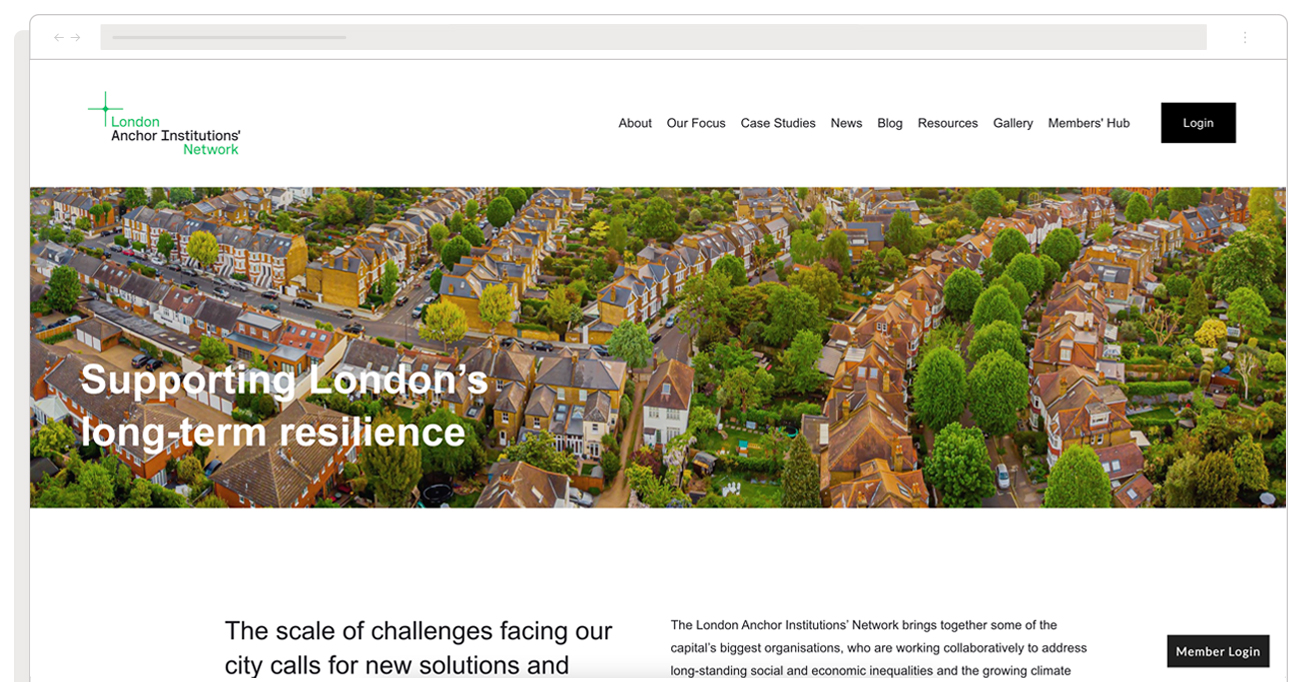The image features a web page layout with a grey outline and a prominent grey box at the top, containing left and right arrows. Below these arrows, a green "X" symbol appears, accompanied by the word "London" in green. The accompanying text includes black font terms such as "anchor," "institutions," and "network."

On the right side of the web page, navigational links include "About," "Our Focus," "Case Studies," "News," "Blog," "Resources," "Gallery," and "Members Hub." Additionally, there's a black box with "Login" in white lettering.

In the main section of the page, aligned to the left, white font text declares, "Supporting London's long-term residents," overlaying a photograph depicting rows of houses surrounded by trees and grey roads. Beneath this, a header states, "The Scale of Challenges Facing Our City Calls for New Solutions," followed by a small black font paragraph that reads: "The London Anchor Institutions Network brings together some of the capital's biggest organizations who are working collaboratively to address long-standing social and economic inequalities in the growing climate."

Adjacent to this paragraph, a black box contains the text "Member Login" in white font. The overall design emphasizes the community-focused mission and collaborative efforts of the London Anchor Institutions Network.